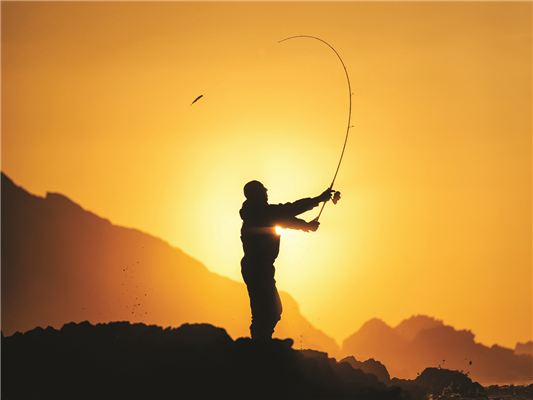In the vertical rectangular image, there is a striking photograph taken during sunrise or sunset, characterized by a diffuse, mustardy orange-yellow glow that bathes the entire scene. Dominating the center of the image is a silhouette of a person—gender indeterminate due to the backlighting—with very short hair or a bald head, facing to the right. Their outstretched arms hold a fishing pole, suggesting they are fly fishing. The fishing pole extends diagonally upward to the right and then curves back to the left, with a fishing line that appears to hang from its tip, though any catch or objects attached to the line are indistinct. 

The silhouette stands atop a landscape feature that is a cross between a low hill and a plateau, covered in dirt clods and rocky terrain. The background features a range of hills and a sloping mountain, creating a layered effect. The two pointed hills to the left stand out against the larger, more gentle slope of the mountain behind the figure, which descends towards a valley before rising again to the right. The sun, partially obscured and appearing as a glowing highlight beneath the person's right armpit, adds to the evocative scene, casting long shadows and enhancing the silhouettes.

The overall aesthetic suggests the image could belong to a travel brochure, a fly-fishing catalog, or an artist’s portfolio, highlighting the beautiful yet stark interplay of light and shadow in a rugged, serene landscape. The quality of the photograph indicates it was taken in the past 20 years, capturing the timeless act of fishing against a breathtaking natural backdrop.